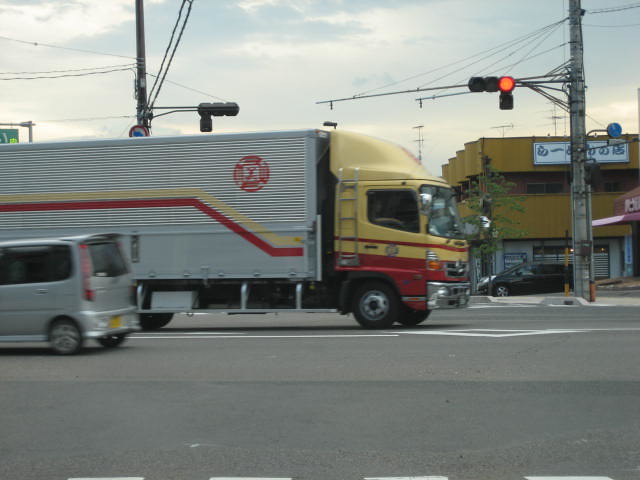The photograph captures a bustling intersection within what appears to be an urban or metropolitan area. Dominating the image is a vibrant semi-truck, with the cab in striking hues of yellow and red. The truck's trailer is primarily white, decorated with horizontal yellow and red stripes and an indistinguishable logo. This semi-truck is crossing the intersection, heading in the opposite direction of a sleek, silver car. Notably, there is also a black minivan in the scene. 

The intersection is governed by an older-fashioned stoplight, which is black and red and attached to a gray pole. The background features several buildings with the most prominent being a gold-colored structure and a partially visible pink edifice. A tree adds a touch of greenery to the setting. The scene is framed by a cloudy, gray sky that hints at impending weather changes. 

The road surface is marked for traffic, and no pedestrians can be seen. The positioning of all elements—the semi-truck centrally located with its trailer extending to the left, the silver car positioned beneath the trailer, and the stoplight and pole in the upper right corner—creates a dynamic snapshot of a routine yet lively city day.